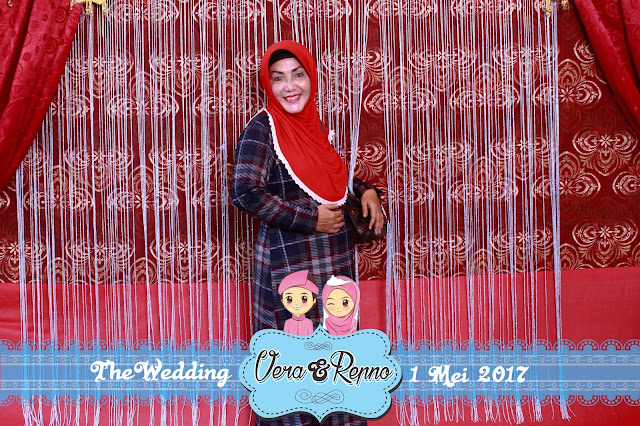A woman, possibly pregnant and wearing a red hijab and a black cap, stands in front of a beautifully decorated backdrop. She has peachy-colored skin and is dressed in a navy blue and red plaid dress, with her hand resting on her stomach in the classic gesture of pregnancy. The backdrop consists of red curtains swept to the sides, with thin white tassels draping down from the top. Behind the tassels, there are intricate patterns of white flowers on a red background. 

At the bottom of the image, a blue light bulb banner stands out, reading "The Wedding" in white font, along with the date "1st May 2017," with the word "May" spelled as "M-E-I." In the middle of the banner, a logo shows a man and a woman, identified as Vera and Reno, who are getting married. The man on the left and the woman on the right are both wearing pink outfits.